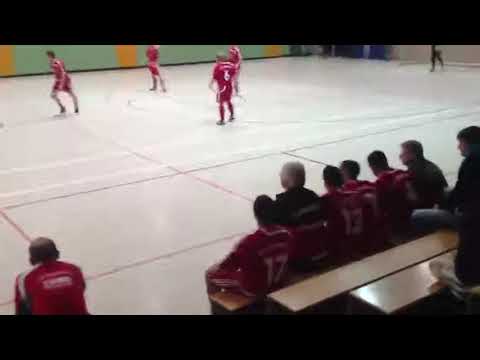This photograph captures an indoor sports game, presumably volleyball or basketball, inside a gymnasium with a light brown, white-lined court floor. Dominating the center are four to five players actively engaged in the game, all wearing red uniforms. The players, appearing Caucasian, wear red shirts and shorts with white print. Surrounding the court, particularly in the bottom right and lower left corners, are several other players and coaches seated on brown bleacher-style benches. These seated individuals are distinguished by their red uniforms and a couple in black jackets who are possibly coaches. The gymnasium features a green back wall accented by three vertical orange stripes. The image has black horizontal strips running across the top and bottom, adding to its somewhat grainy and dark quality. The scene is devoid of textual elements, with a color palette including red, white, black, tan, silver, gray, yellow, green, and blue.